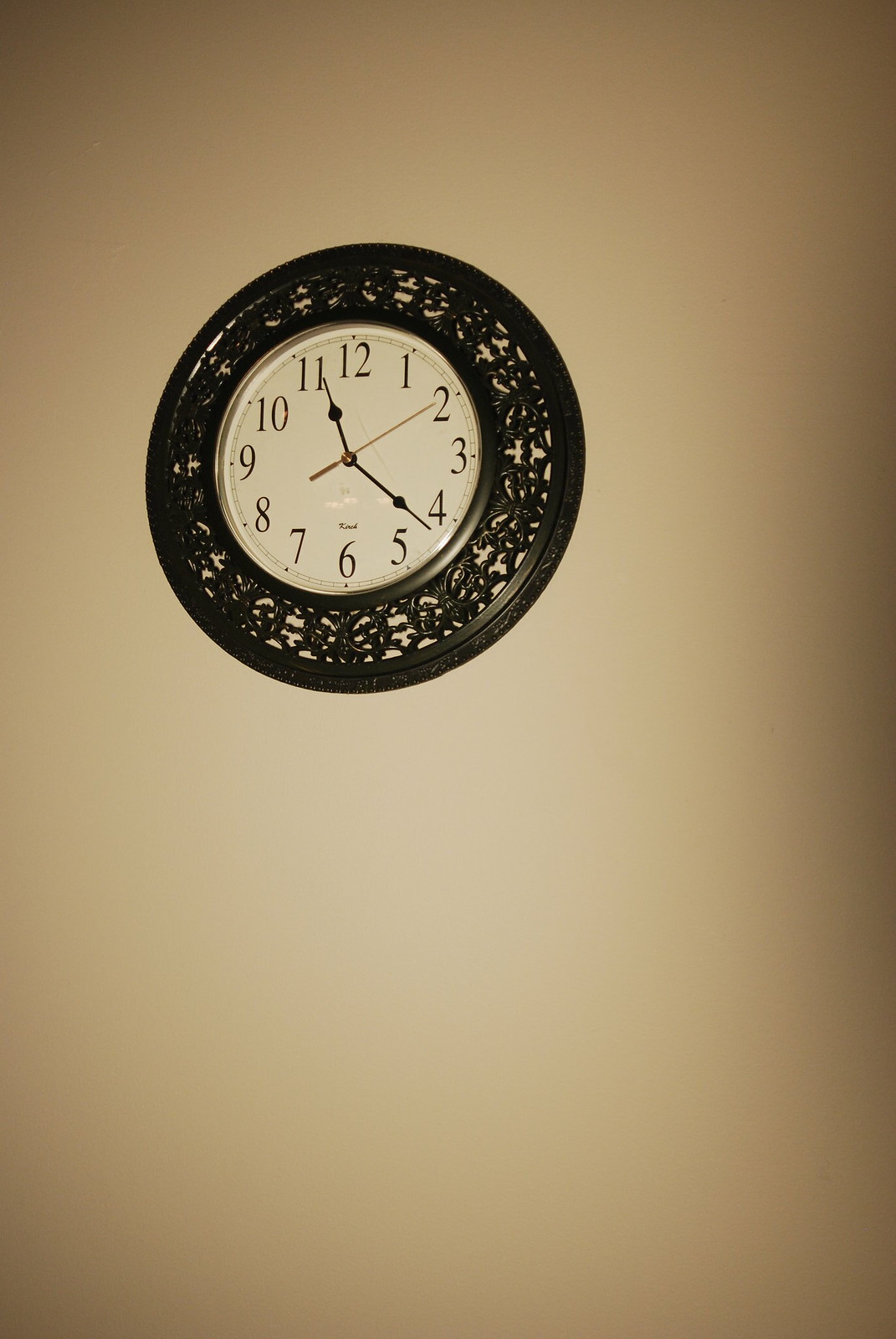This photograph captures a small, round wall clock with a strikingly ornate black border adorned with intricate decorative designs. The clock face is a pristine white, providing a clear contrast to the elegantly simple numerals which lack any stylization, ensuring easy readability. It features three hands: the hour and minute hands are black, while the second hand, which is particularly thin, is brown. The time displayed is a little past 11:20. The background of the image is a soft, light beige color, which subtly complements the clock's design, highlighting its aesthetic details.